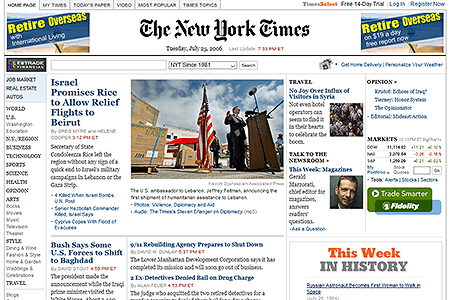This image, sourced from the New York Times online edition, is dated Tuesday, July 25th, 2006, with a last update timestamp of 7:33 PM displayed in red. The iconic New York Times masthead, featuring elaborate calligraphy-style lettering, is prominently visible at the top. The page highlights several major news articles. One headline reads, "Israel Promises Rice to Allow Relief Flights to Beirut," indicating a diplomatic effort related to the Israeli conflict. Accompanying this article is a photograph that includes the American flag and an interview scene, set against a backdrop of large containers, likely housing the relief supplies such as rice.

Another significant headline reads, "Bush Says Some U.S. Forces to Shift to Baghdad," reflecting military strategy updates during the Iraq War. Additional articles are also featured: "This Week in History," and "No Joy Over Influx of Visitors in Syria," providing historical context and regional news. Additionally, the page includes sections on opinions and market updates. The detailed layout combines text and images, offering a comprehensive snapshot of global and political events at the time.